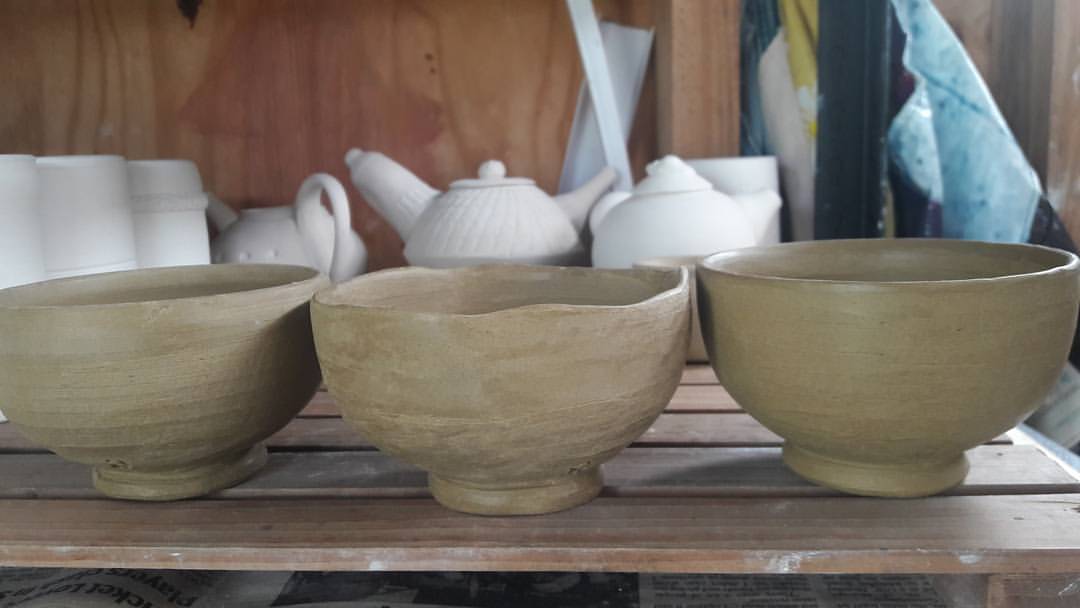The photo is a color image taken inside a pottery studio. In the foreground, three bowls crafted from gray clay sit on a drying rack made of thin boards with gaps to allow for airflow. These bowls appear to be the work of a beginner, with the ones on either side showcasing a round, well-formed shape with a foot, while the bowl in the middle features a distinct wavy edge at the top, possibly a deliberate artistic choice. All three bowls seem wheel-thrown rather than coil-made and are at the leather-hard stage, where they are not yet fully dry but are firm enough to trim.

Behind the gray bowls, on an upper shelf, there are several white bisqueware pieces that have already been fired once. Among these are various teapots, some with looped handles, others with straight handles, indicating different styles and techniques. Other pottery items, possibly inverted forms or vases, are also on this shelf and appear ready to be glazed. The area is framed by a plain plywood wall in the background, with what looks like smocks hanging on the upper right side. The workspace is clearly a functional and active pottery studio, with different stages of pottery making on display.